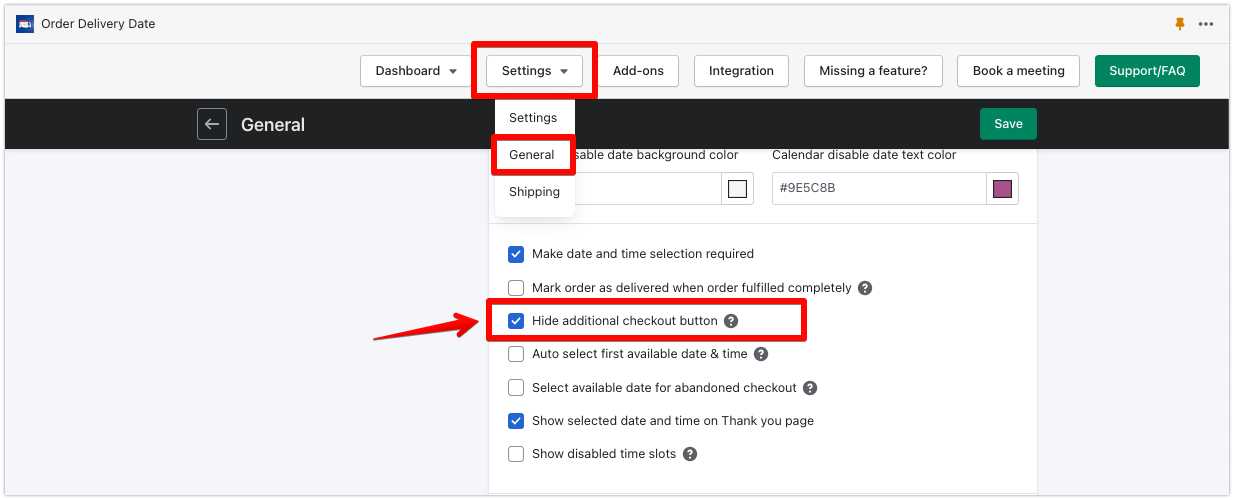This image is a detailed screenshot of a website interface displayed against a light gray background. In the top left corner, there's a dark blue square containing a cartoon graphic of a van. Adjacent to this graphic is the phrase "Order Delivery Date" with the letters 'O,' 'D,' and 'D' capitalized in black text.

To the right of this area, there is an orange pushpin icon pointing downwards, next to which three circles are aligned side-by-side. Below this, near the center of the screenshot, are various navigational options. The first option is labeled "Dashboard" with a drop-down menu. The second option, "Settings," is surrounded by a red border. The "Settings" option also includes a drop-down menu, with sub-options such as "General," which also has a red outline, and "Shipping."

Further to the right of these settings, the options listed are "Add-ons," "Integration," "Missing a Feature," "Book a Meeting," and finally, a green tab labeled "Support/FAQ" in white text.

Towards the bottom of the screenshot, there is a black banner with a white outline of a square containing a left-pointing arrow. Outside of this square, the word "General" appears in white text. On the far right, a green tab with white print says "Save."

In the central area of the screenshot, a gray background is marked with a white square containing various settings options. These include: "Disable the background color," "Calendar Date," "Disable the text color," "Mark date and times required," and "Mark order as delivered when fulfilled completely." A red square or outline highlights the option "Hide additional checkout button" with an arrow pointing at it. Additional settings include "Auto-select first date and time," "Select available date for abandoned checkout," "Show select a date/time on the Thank You page," and "Show disabled time spots."